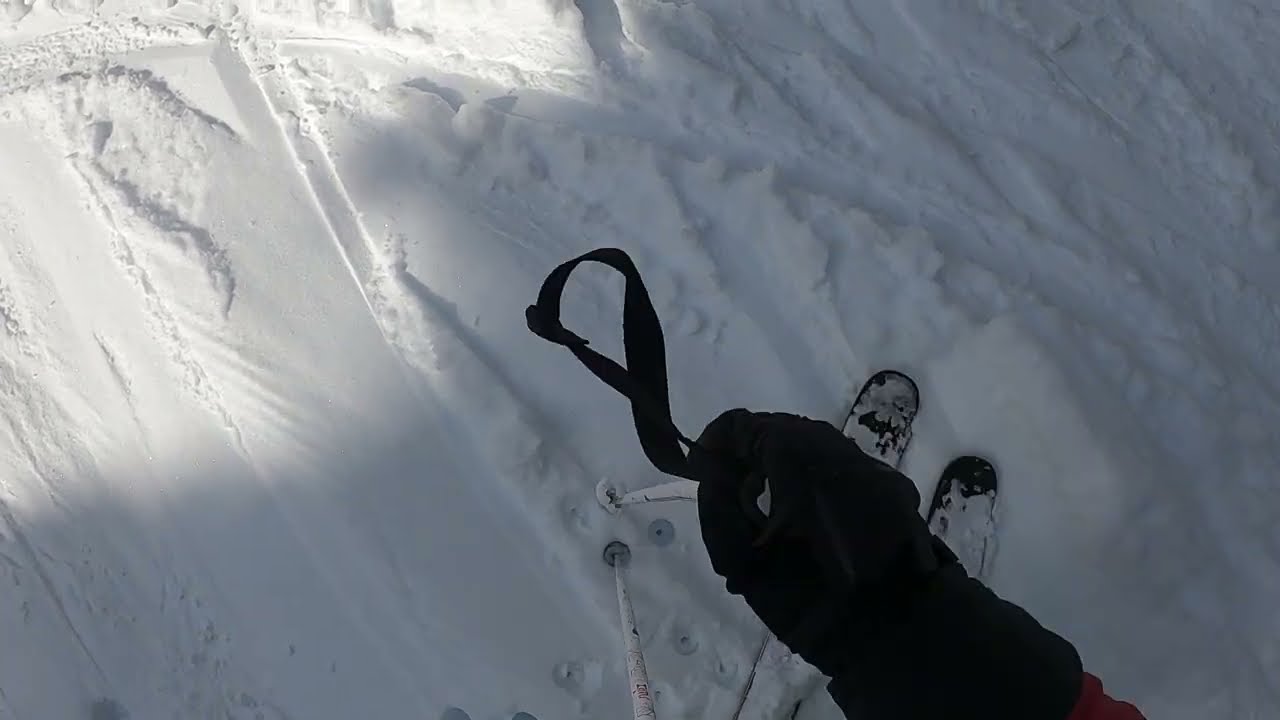This dynamic photograph, likely taken from a GoPro mounted on a skier's helmet, captures an action-packed skier's-eye view of a snow-filled trail. The frame is predominantly filled with snow, showcasing various ski tracks and markings from previous adventurers. Centered at the bottom of the image, a pair of skis, distinct with their black edges dusted with white snow, protrude into view, alongside two thin white ski poles. A single black-gloved hand grips one of the poles, adding a sense of movement and human presence. The majority of the scene is shrouded in shadow, contrasting with the top left corner where the sun brilliantly illuminates the snow, casting a bright, reflective glow. The captivating mix of light and shadow accentuates the texture of the snow and the skier's gear, immersing the viewer in the thrilling perspective of a downhill ski run.